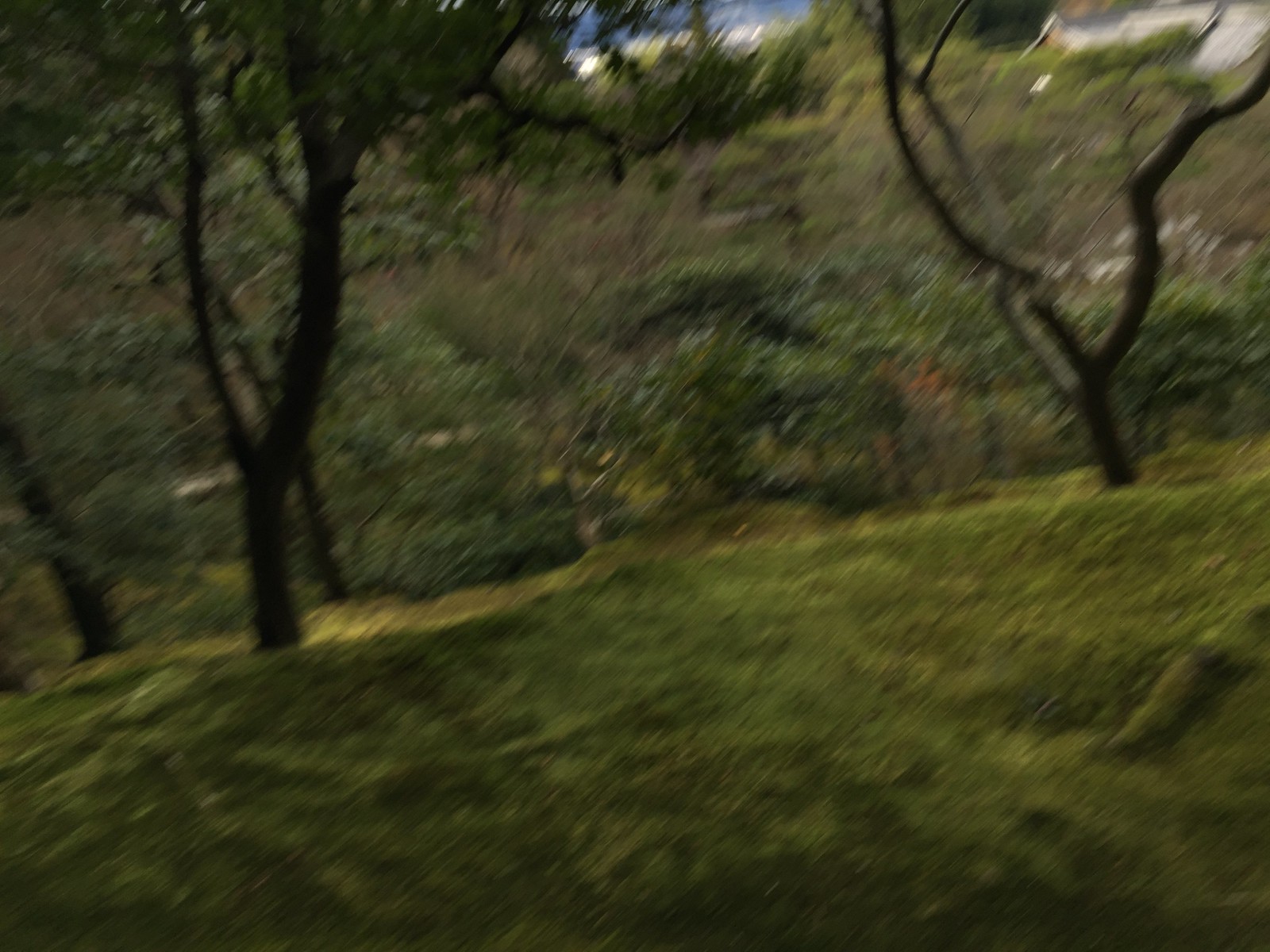This photograph, though slightly blurry, offers a captivating glimpse into a verdant wooded trail, likely a popular hiking path. The lush green grass dominates the foreground, creating an inviting entrance to the trail. Flanking the pathway are two mature, robust trees—one on the left and another on the right—emphasizing the dense and thriving nature of the forest, which suggests it is late spring or summertime. The backdrop is a picturesque grove of trees and various vegetation, bursting with different hues. In the distance, gentle hills rise, creating a sense of depth and adventure. The sky above is mostly clear, with a scattering of small clouds, adding to the tranquil ambiance of the scene. Despite its slight blurriness, the photograph vividly conveys the natural beauty of the hilly area and its striking vegetation.